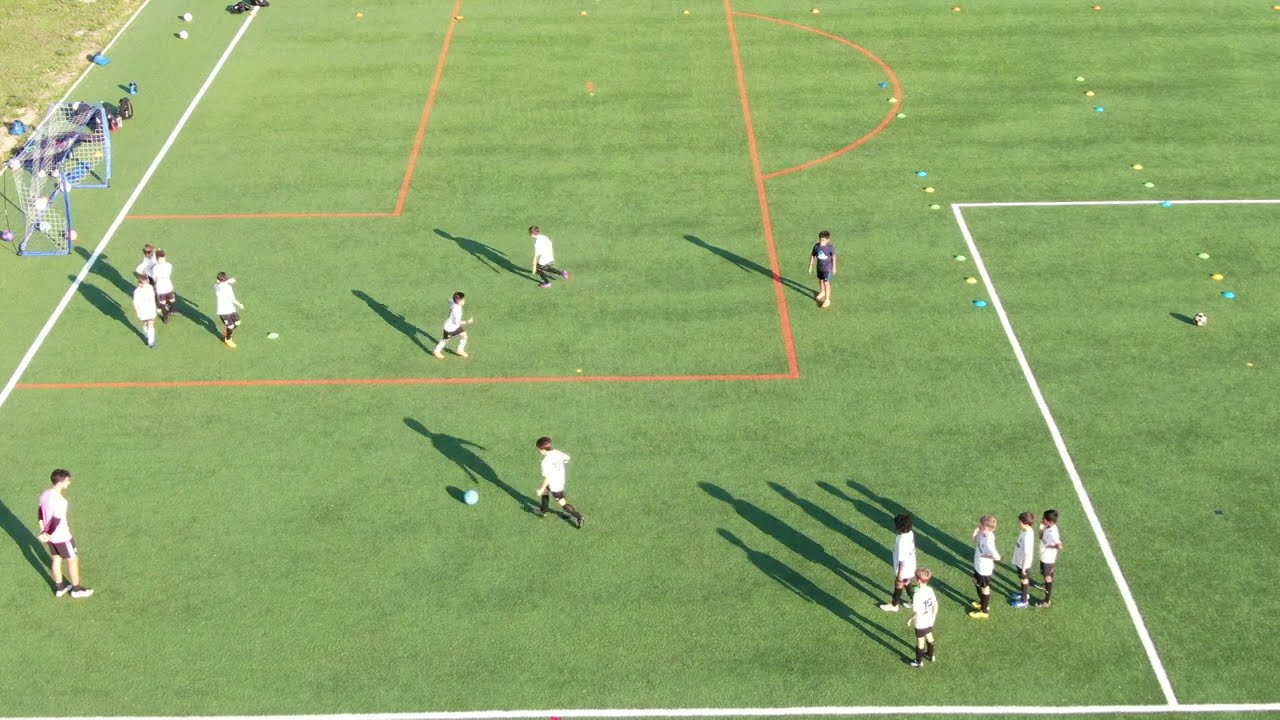The image depicts a vibrant, daylit scene of a children’s soccer practice taking place on a well-maintained green grass or AstroTurf field. The bright daylight illuminates the scene, casting long shadows from right to left, enhancing the visibility of the children’s activities. At the bottom of the photo, children dressed uniformly in white shirts and black shorts line up, taking turns to kick a ball towards the goal. An adult coach, located in the bottom left corner, closely supervises the kids. He has brown hair, Caucasian skin, and wears a white short-sleeved shirt over a long-sleeved black one, paired with black shorts. In the lower right corner, a group of five children waits eagerly for their turn. The field markings are quite distinct, with a white line running at a 90-degree angle towards the top corner and a red line resembling a basketball court shape, adding further details to the setup. There’s a sprinkling of more children practicing in the middle of the field, creating a lively and dynamic atmosphere as they all cast long shadows to the upper left of the frame, emphasizing the practice setting of this engaging sports moment.